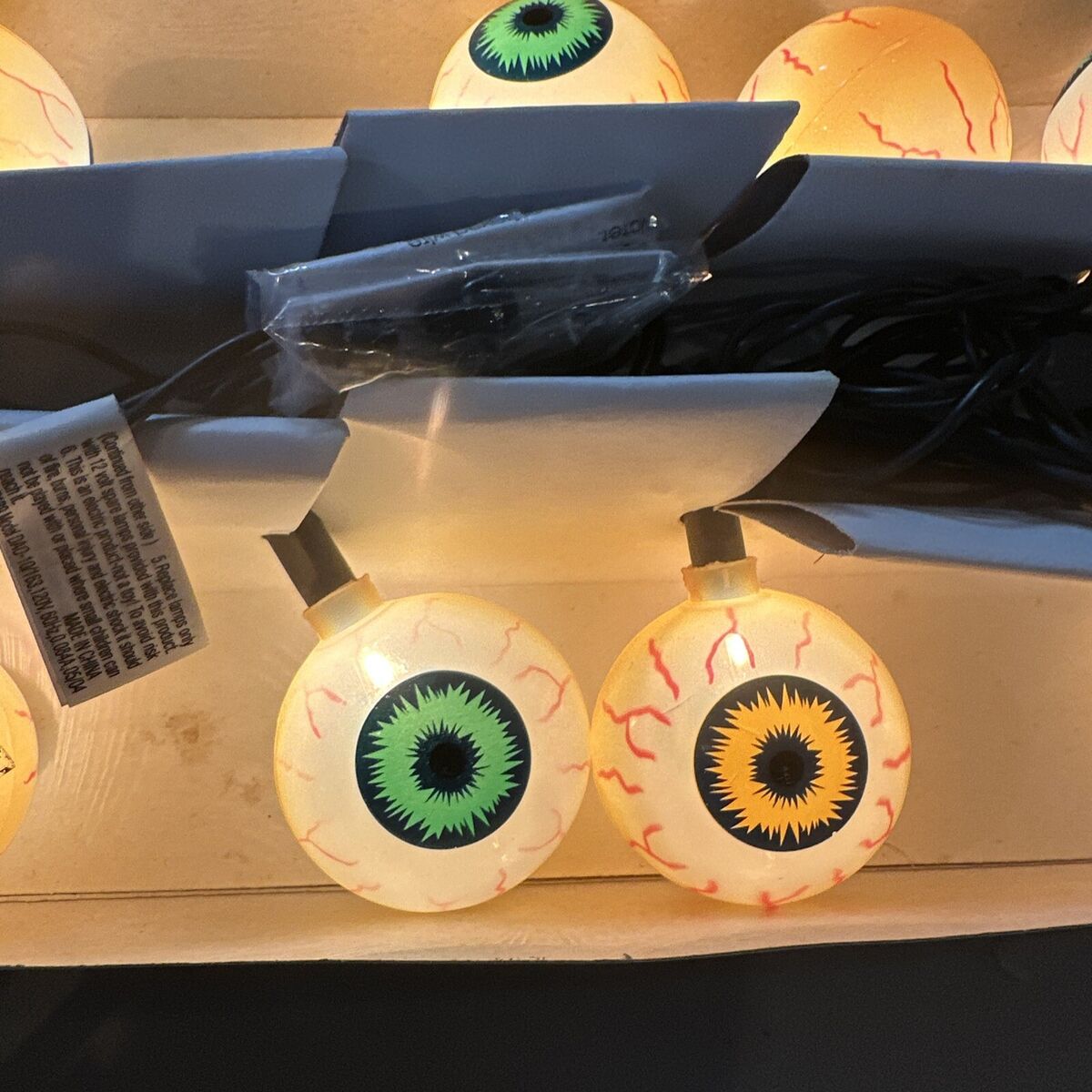The image displays a set of eerie, glowing light bulbs designed to resemble bloodshot eyeballs, likely intended as Halloween decorations. The central focus is on two eyeball-like light bulbs: the left one features a creepy green iris, while the right sports an ominous orange iris. Both are set against a white sclera, streaked with red, blood vessel-like markings that give a strained, lifelike appearance. A third eyeball light with a green iris is partially visible at the top, and a fourth eyeball is seen from behind, showcasing only its cream-colored backside adorned with red squiggles.

Above these two central eyeballs, there's an organizational structure, possibly a packaging unit with slits designed to hold the cables of these spooky lights. The packaging is light blue and has black cords extending from it, one of which features a tag with indistinct writing. Higher up, another similar organizer is in place, with additional eyeball lights partially visible, gazing in various directions, enhancing the unsettling atmosphere of the image.